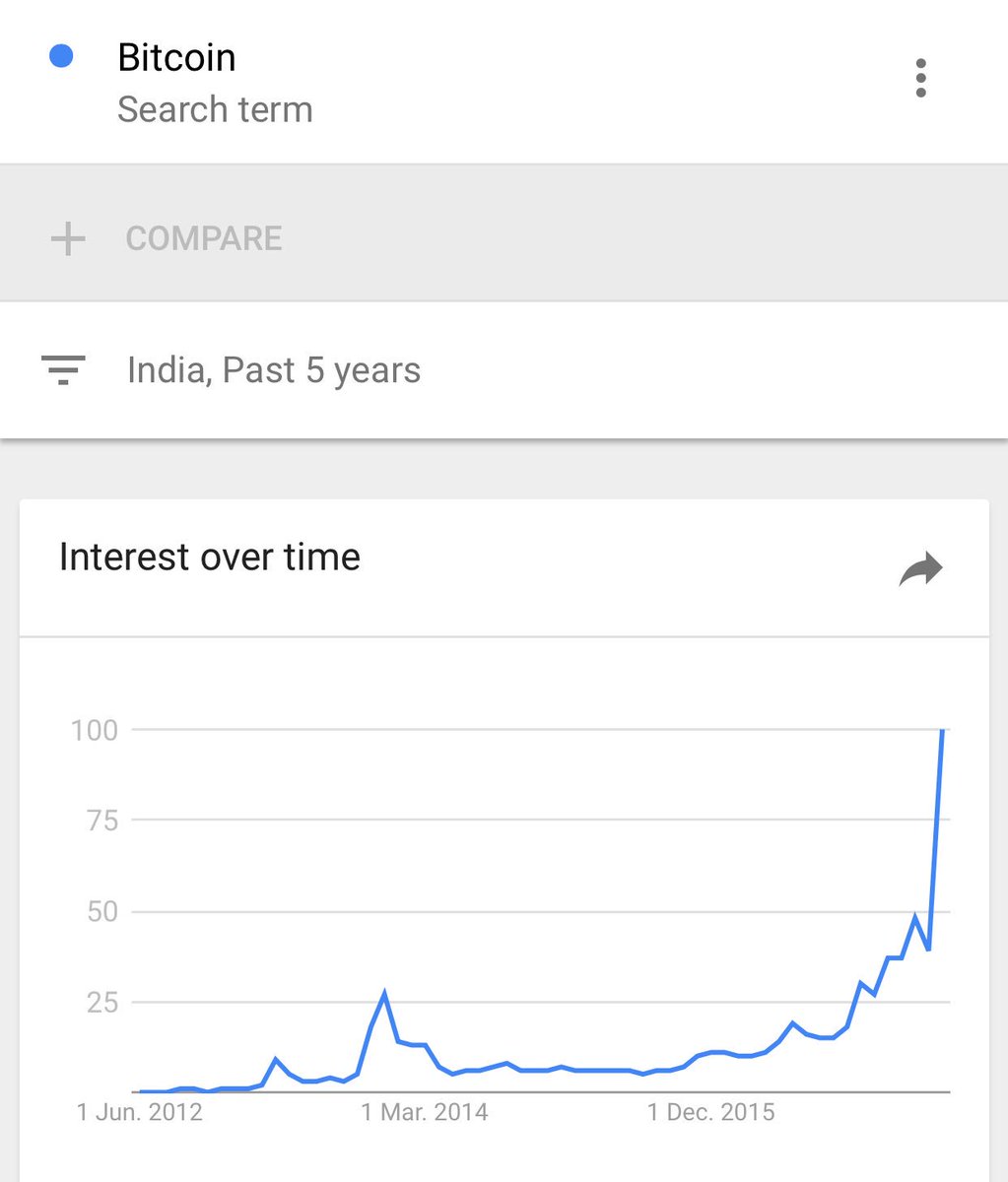The image features a Bitcoin-related website with the word "Bitcoin" prominently displayed at the top in black text, accompanied by a blue dot beside it. There is a search term input field and a three-dot menu on the right-hand side of the header. Below this section is a gray horizontal bar that spans the width of the page. This bar includes a plus sign, the word "Compare" in gray text, and text that reads "India, past five years."

Within the gray bar, there is a smaller white box containing the text "Interest over time," and an arrow pointing to the right. Below this, there is a gray line graph with vertical markers in increments of 25, labeled from 0 to 100, to indicate varying levels of interest. The x-axis displays a timeline from June 2012 to December 2015.

The line graph illustrates fluctuating interest levels in Bitcoin over time, starting with lower, irregular values between June 2012 and December 2015. After 2015, the graph shows a marked increase in interest, culminating in a peak that reaches the 100 mark on the scale.